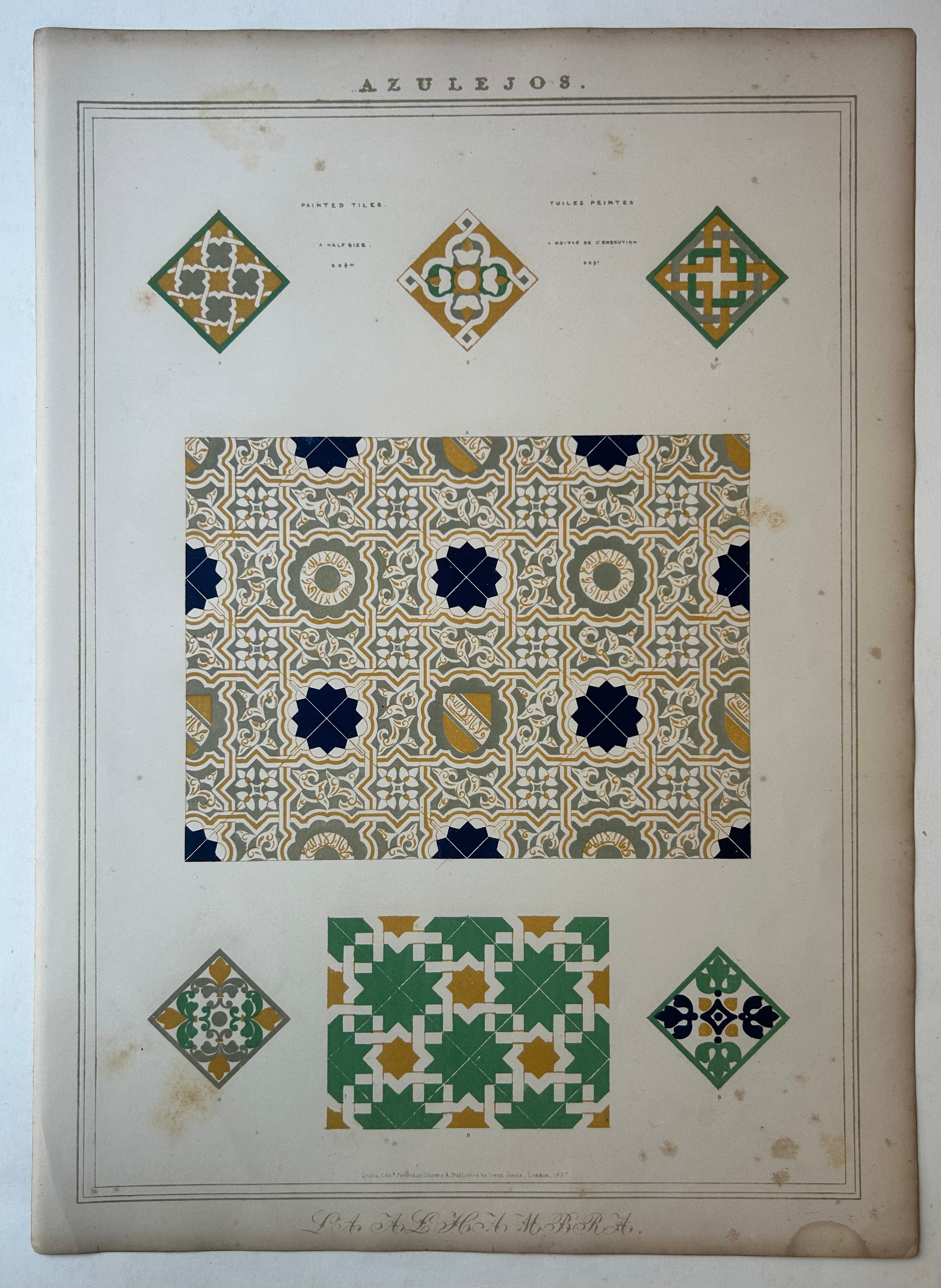This image is an old, faded page, possibly from a catalog or book focused on intricate patterns, likely tile designs, and possibly of Spanish origin. The page, titled "Azulejos" in ornate calligraphy that is difficult to decipher due to age and water stains, features a variety of geometric and floral designs that are richly detailed. At the top of the page are three primary patterns displayed in diamond shapes. The first pattern features yellow X's within gold squares, the second pattern is a gold-outlined cross, and the third combines gold, green, and blue in an interwoven cross design. Below these, centrally, is a square with complex shapes in blue, gray, and yellow, offering a striking composition on a white background. Towards the bottom, there are additional patterns: a green and gold diamond flank on either side of a smaller green and mustard yellow rectangle. The whole page is bordered, encapsulating these vibrant, yet faded designs, capturing the essence of elegant, historical tile patterns in a meticulously illustrated and timeless manner.